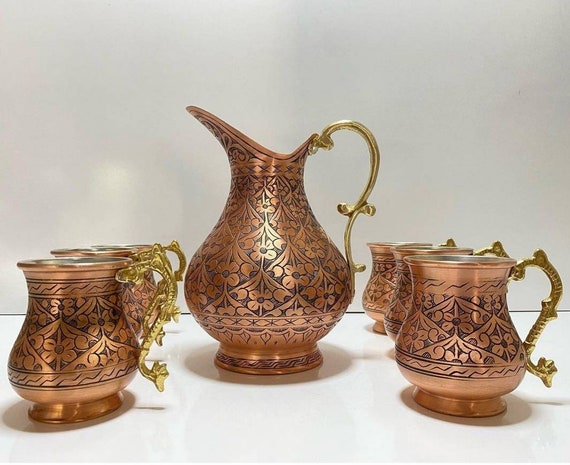In this photograph, a beautifully elaborate tea set is showcased, consisting of a central copper jug flanked by six copper cups, three on each side. The jug features a striking gold brass handle that curves elegantly, mirrored by the similarly curved handles on the cups. A consistent floral pattern, resembling flower petals, intricately decorates both the jug and cups, creating a harmonious design. The jug and cups also include delicate etchings that give a detailed yet simple appearance. The set, with its ornate craftsmanship, suggests origins from cultures known for elaborate metalwork, possibly Turkish or Indian. The entire arrangement is displayed on a white surface with a pale gray background, highlighting the warm tones of the copper and gold.